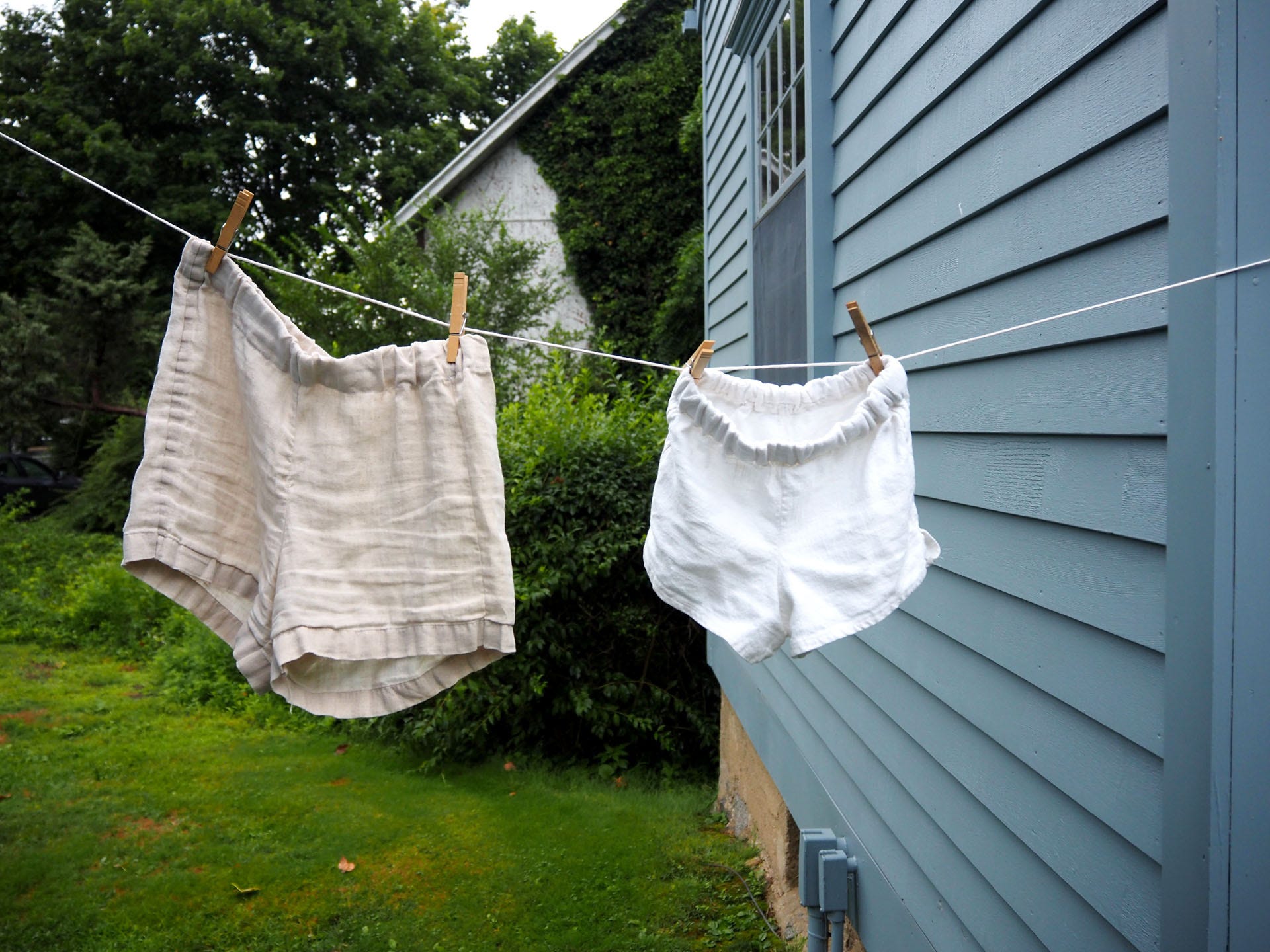In this landscape-oriented real-life photograph, a simple domestic scene is vividly captured. The main focus is a thin white washing line stretching horizontally across the center of the image, bearing two pairs of shorts secured with wooden clothespins. The left pair of shorts is an off-white/tan color, likely belonging to an adult, characterized by an elastic waistband hinting at comfort and casual wear. The right pair, smaller and purely white, likely belongs to a child, also featuring an elasticated waistband.

Behind the smaller white shorts, the siding of a house provides a backdrop. The house has a horizontal turquoise-blue paneling and features a single window with a tinted upper glass pane and a mesh lower section, reflecting some light. Below the blue siding, the base of the house is an earthy tan color with two entry ports, possibly for utilities or piping.

On the left side of the image beneath the larger shorts, a patch of green grass is visible, interspersed with bare patches of brown dirt and scattered leaves, indicating a well-used yard. In the background, a lush setting of shrubs and trees offers a sense of seclusion, with larger trees forming a natural canopy behind the scene. Partially obscured by foliage, the pitched roof and a white section of another property peek through on the right, adding to the layered depth of the image.

Overall, the photograph emphasizes a serene, everyday moment of life at home, capturing the simple act of hanging laundry against a backdrop of natural and structural elements.